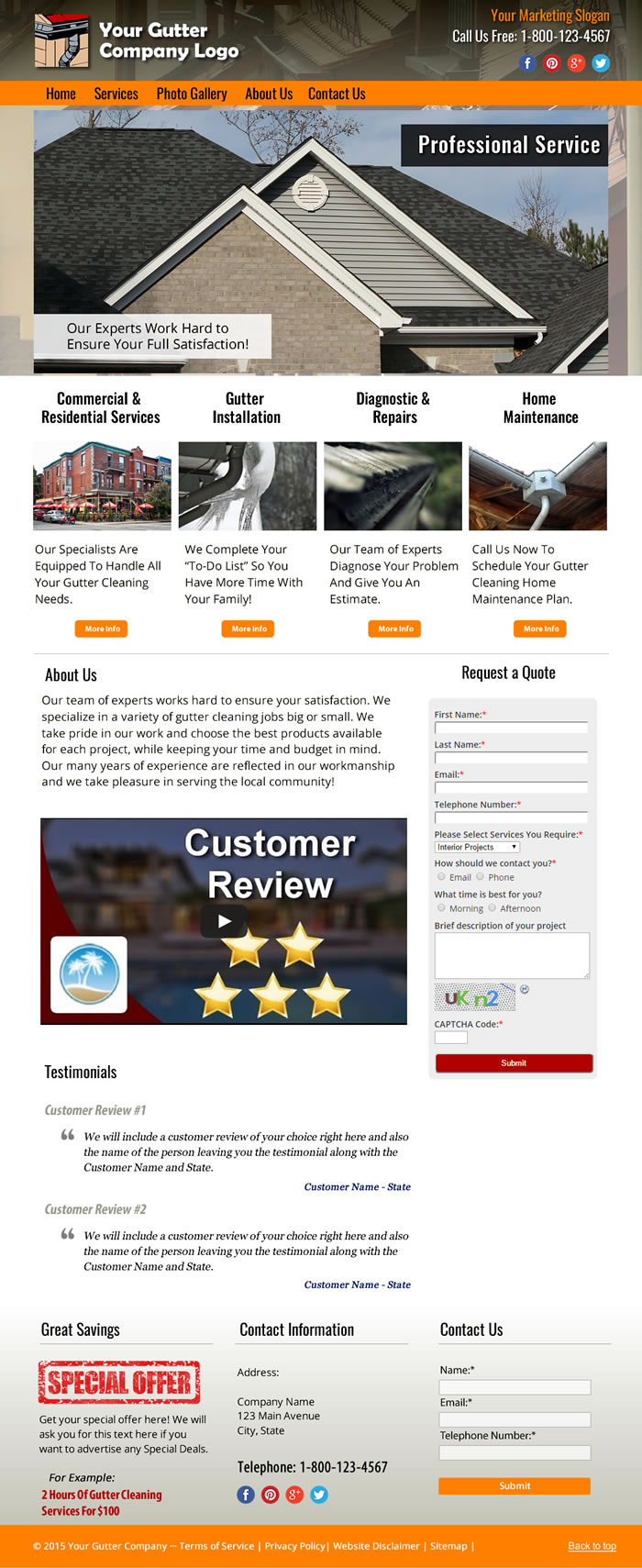The image displays a well-organized layout for a gutter company's website. At the top, there is a border featuring the company's logo, with phone numbers and social media icons neatly positioned to the right. Below this, an orange menu bar provides navigation options, including "Home," "Photo Gallery," and "Contact Us," though the text appears small and slightly difficult to read.

Directly beneath the menu bar is a prominent image of a house, accompanied by a caption that reads "Professional Service" against a boxed background. Further down, there is a section labeled "Customer Review" that highlights a five-star rating in gold. To the right of this section, a box titled "Request a Quote" includes fields for users to input their information, along with a CAPTCHA to complete.

At the bottom of the layout, a gray area features a red label on the left side that says "Special Offers," followed by additional text boxes for contacting the company. This detailed organization ensures that all essential information is easily accessible to the user.